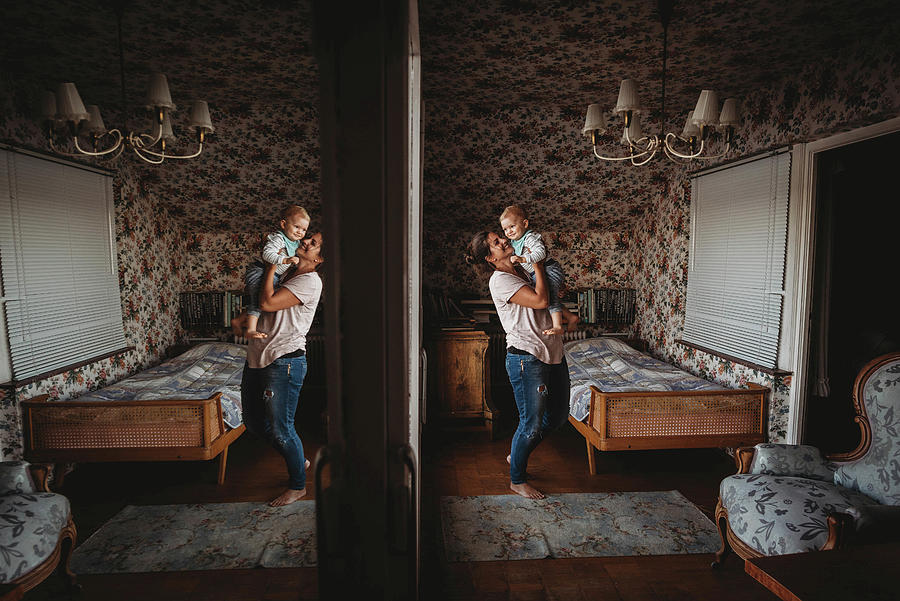In this intriguing image, a young woman in a white t-shirt and blue jeans is holding her baby above her head in a narrow bedroom, creating a nostalgic and vintage ambiance. Remarkably, the picture is split into two symmetrical halves, revealing two perfectly mirrored rooms. On the right side, the woman faces right, lifting her baby who is glancing leftwards, dressed in a light blue shirt and blue shorts. The backdrop features a wicker bed with a blue cover, a wooden floor with a small area rug, and furniture adorned with numerous books. Floral wallpaper in shades of light and dark brown envelops the room, accented by a hanging chandelier and white window blinds. In the mirrored left side, the woman now appears on the left, maintaining the same pose and expression. A large, open doorway introduces a sense of depth, while a chair with a blue cushion and brown borders sits prominently in the corner. The overall aesthetic, combining hues of brown and light blue, along with dense floral patterns, evokes an old-time charm.